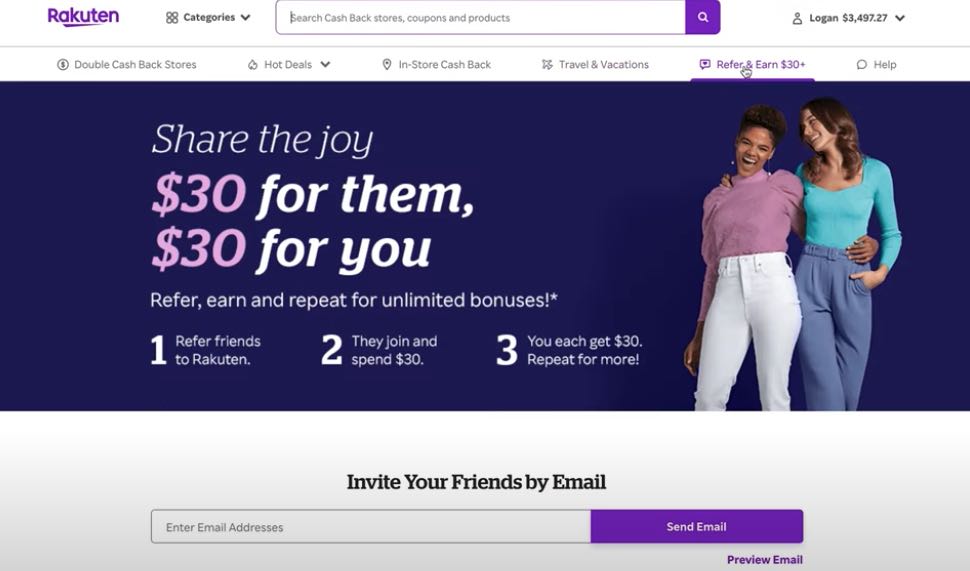A detailed screenshot of a Rakuten website displayed on a desktop or laptop browser. In the top left corner, the Rakuten logo is prominently visible in purple text with a distinctive purple dash underneath – spelled R-A-K-U-T-E-N. At the very top is a purple search bar with the text: "Search cash back stores, coupons, and products." To its left is a drop-down menu labeled "Categories." On the right, the current logged-in account is identified as "Logan," alongside an impressive balance of $3,497.27.

Beneath the header, there’s a navigation bar with multiple tabs: "Double Cash Back Stores," "Hot Deals," "In-Store Cash Back," "Travel and Vacations," "Refer and Earn $30," and "Help." The cursor is currently hovering over the "Refer and Earn $30" tab, highlighted in purple.

Below this bar is a banner image featuring two women joyfully holding each other and smiling, both dressed in long-sleeved shirts and pants of different colors. To the left of the image, text reads "Share the joy $30 for them, $30 for you." Further down, it states "Refer, earn, and repeat for unlimited bonuses," followed by a brief three-step referral process. There is an invitation to "Invite your friends by email" with an email address entry field. To the right is a purple "Send Email" button. Below this button, a purple text link states "Preview Email."